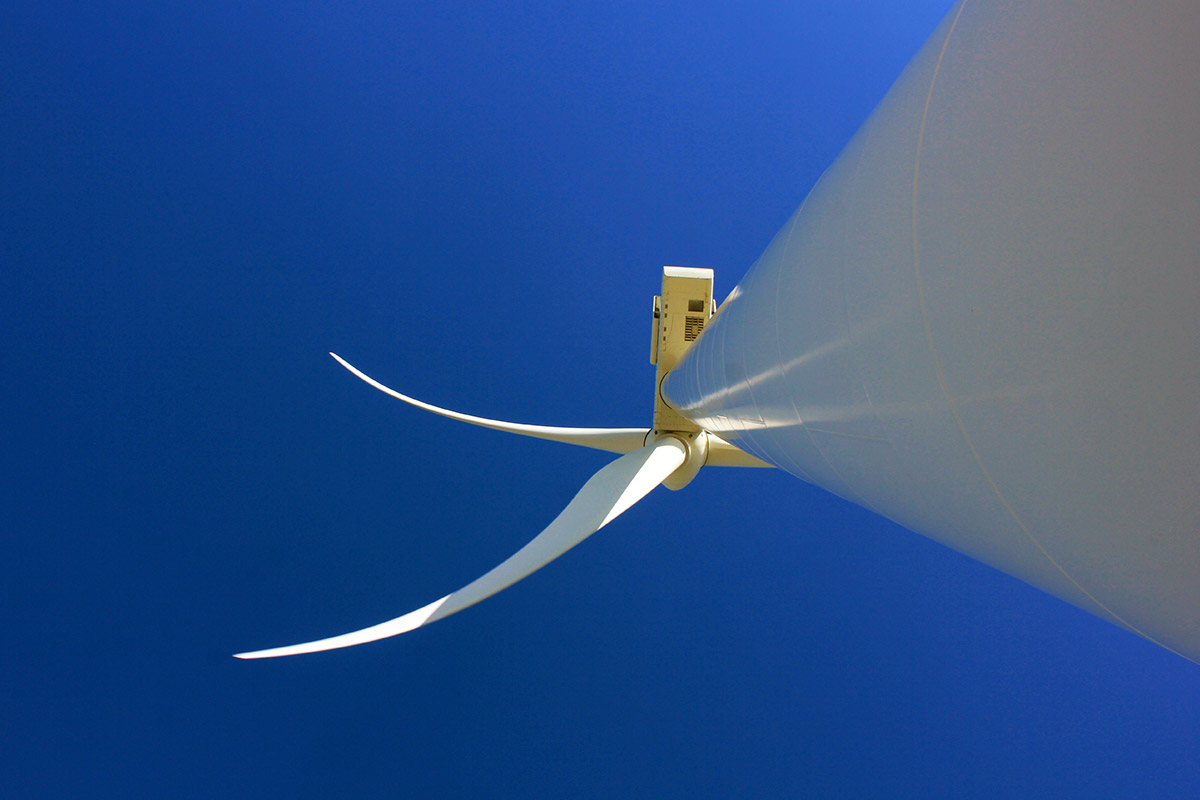The image features a towering wind turbine photographed from its base, looking straight up along its white or grayish shaft, which stretches diagonally from the top right to almost the bottom left of the frame. The sky in the background is an extraordinarily bright, crystalline blue, so vivid it almost seems surreal. Dominating the right side of the image, the robust pole supports a metal-encased motor at its summit. From this motor, three large, curved blades extend outward, forming a striking visual against the blue sky. The perspective and composition emphasize the height and grandeur of the turbine, making the viewer feel as though they are standing right beneath this modern marvel of engineering.